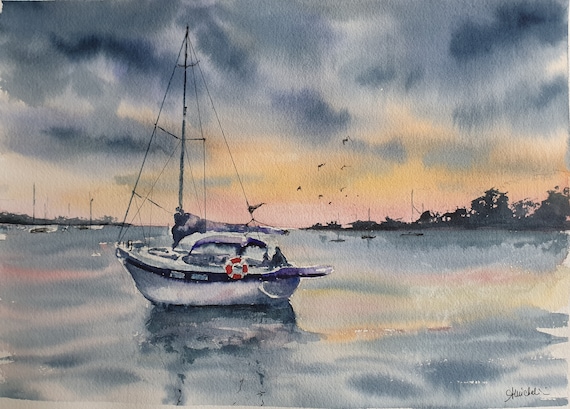This detailed watercolor painting depicts a small white sailboat with navy blue accents and a visible mast, prominently centered on a serene body of water. The boat features a red and white lifesaver hanging from its side. Above, the sky is a mix of dark clouds with orange, pink, and gray hues, suggesting the cusp of sunset or sunrise. The water mirrors the sky's colors with less intensity in its shades of gray. In the background, more sailboats dot the horizon along with glimpses of distant land and trees. Birds can be seen flying amidst the cloud-filled sky, adding to the tranquil yet dynamic scene.